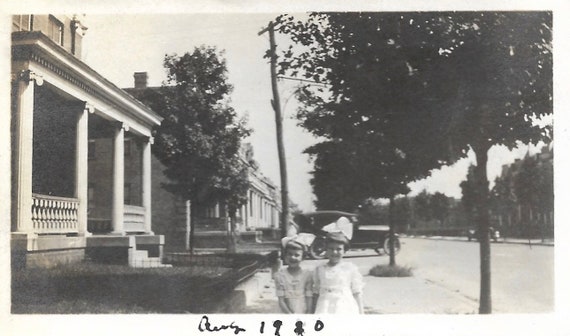This black-and-white photograph, dated "AUG 19," likely from the 1920s, features two young girls in the foreground, perhaps sisters, standing on a neat sidewalk. They both wear short hair with bangs, immaculate white dresses, and large, fluffy white bows atop their heads. To their left is a grand two-story house adorned with a spacious porch supported by white columns, accessed via brick and concrete steps. To their right, a tree-lined street extends, creating a picturesque, shaded scene. Behind the girls is an early 20th-century car, possibly a Model T, with an adjacent telephone pole just visible. The background reveals more stately buildings and additional tree-lined sidewalks, capturing a charming, historic neighborhood.